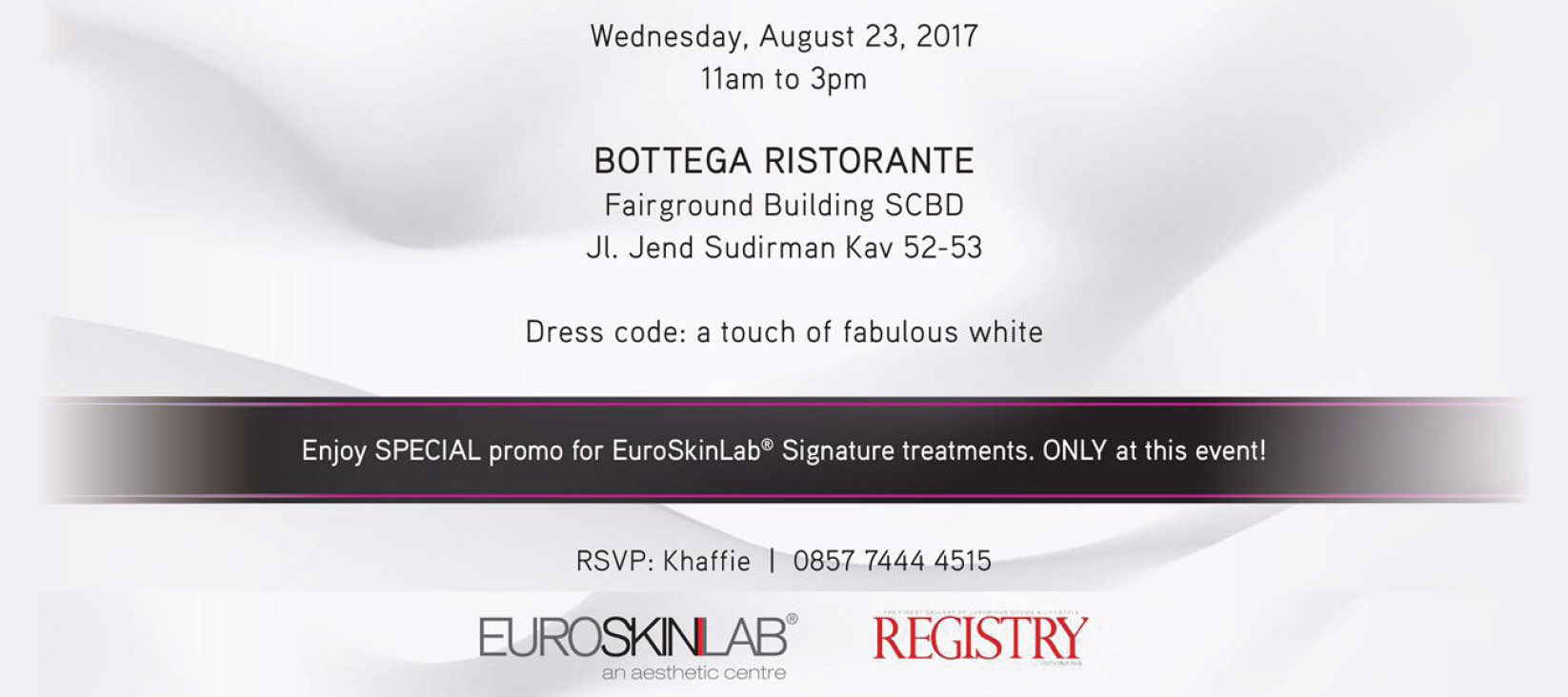This horizontal, rectangular advertisement features a textured white background with a dark, prominent horizontal banner running across the middle. Inside this banner, with stark white text, it announces: "Enjoy special promo for Euro Skin Lab signature treatments only at this event." 

The event information is clearly stated above the banner in smaller black letters: "Wednesday, August 23rd, 2017, 11 a.m. to 3 p.m." In larger black text, it names the venue: "Bottega Ristorante." Below that, in smaller lettering, it lists: "Fairground Building, SCBD, J.I. Gend, Serdiman CAV 5253."

Additional details include the dress code, specified in smaller print: "Dress Code: A touch of fabulous white." The overall color scheme of the image incorporates shades of white, gray, black, purple, and red, giving it a sleek, modern aesthetic. The text is centrally placed, making the advertisement visually balanced and easy to read, highlighting the promotional event for Euro Skin Lab amidst a minimalistic yet textured background, resembling clouds.